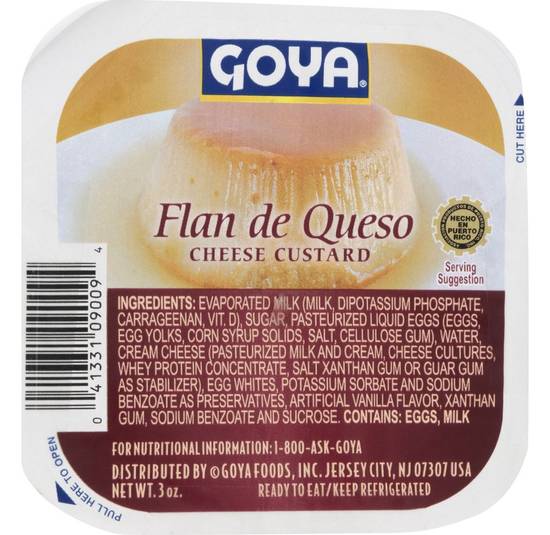This is a photograph of a supermarket product labeled Flan de Queso Cheese Custard by Goya. The product is packaged in a white, rounded square plastic container. The label prominently features a semi-circular white plate with an image of an overturned, cooked custard, accompanied by the product name "Flan de Queso Cheese Custard" in maroon lettering on a yellow background. To the right of the title is a gold seal, and above the flan image, on a blue background, is the recognizable Goya logo in white letters.

The lower half of the label transitions to a maroon background, detailing the ingredients: evaporated milk, milk, dipotassium phosphate, carrageenan, vitamin D, sugar, pasteurized liquid eggs, eggs, egg yolks, corn syrup solids, salt, cellulose gum, water, cream cheese, pasteurized milk and cream, cheese cultures, whey protein concentrate, stabilizers (xanthan gum or guar gum), egg whites, preservatives (potassium sorbate and sodium benzoate), artificial vanilla flavor, and sucrose. It also states "Contains eggs, milk."

Below the ingredient panel is a section providing nutritional information contact details (1-800-ASK-GOYA) and distribution information: Goya Foods Inc., Jersey City, New Jersey, 07307, USA. The packaging specifies "Ready to eat, keep refrigerated" and includes a net weight of 0.3 oz.

On the left side of the container, there is a black-and-white UPC barcode, with a blue arrow and instructions to "Peel here to open" located on the bottom left. Additionally, there is a note at the top right corner instructing to "Cut here."

Overall, the packaging combines clear branding, detailed ingredient lists, and user-friendly opening instructions.